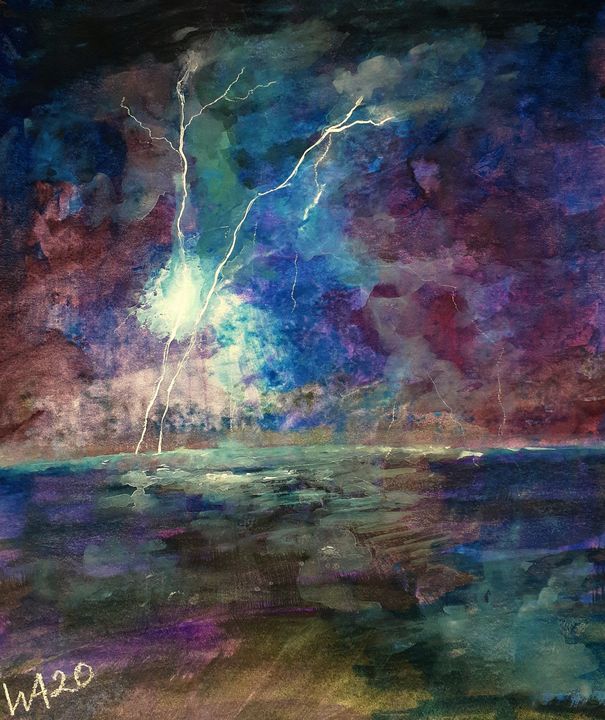The image appears to be a painting set against a murky blue or purple backdrop, imbued with a mix of dark and vibrant colors including dark blue, dark purple, dark red, and dark green. Strewn across the sky are streaks of white lightning, branching out as it ascends or descends, possibly striking or emerging from an indistinguishable object beneath. The backdrop is punctuated with hazy purple markings, enhancing the mysterious, ethereal ambiance. Both the ground and sky feature an array of colors—brown, green, blue, gray, purple, burgundy, beige, and white—creating a complex tapestry of shades and tones. Notably, in the bottom left corner, the artist's signature "WA20" is prominently displayed, offering a modest clue to the creator of this enigmatic and atmospheric piece.